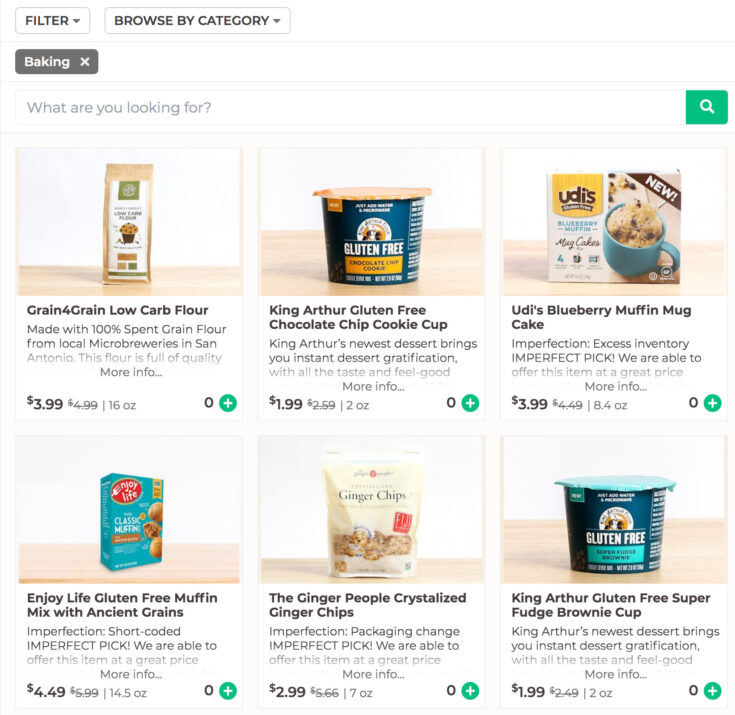The website showcases a selection of baking products for sale. At the top of the page, a white background features gray-outlined boxes labeled "Filter" and "Browse by Category," both with drop-down menus. A gray tag with white print reads "Baking." Below this, a search bar asks, "What are you looking for?" with a green button on the right featuring a white magnifying glass for searching.

The product display includes six items:

1. **Grain-for-Grain Low-Carb Flour**: A brown bag with a white label. Priced at $3.99 for 16 ounces.
2. **King Arthur Gluten-Free Chocolate Chip Cookie Cup**: Packaged in a blue container with an orange top, priced at $1.99 for 2 ounces.
3. **UD's Blueberry Muffin Mug Cake**: Presented in a blue mug with cake inside, displayed in a white box. It costs $3.99 for 8.4 ounces.
4. **Enjoy Life's Gluten-Free Muffin Mix with Ancient Grains**: Packaged in a blue box with a red and white label, priced at $4.49 for 14.5 ounces.
5. **The Ginger People Crystallized Ginger Chips**: Found in a yellow and white bag, priced at $2.99 for 7 ounces.
6. **King Arthur Gluten-Free Super Fudge Brownie Cup**: A blue cup with a teal blue lid, priced at $1.99 for 2 ounces.

Each item features a green circle with a white plus sign in the bottom right-hand corner, indicating the option to add the product to the cart.